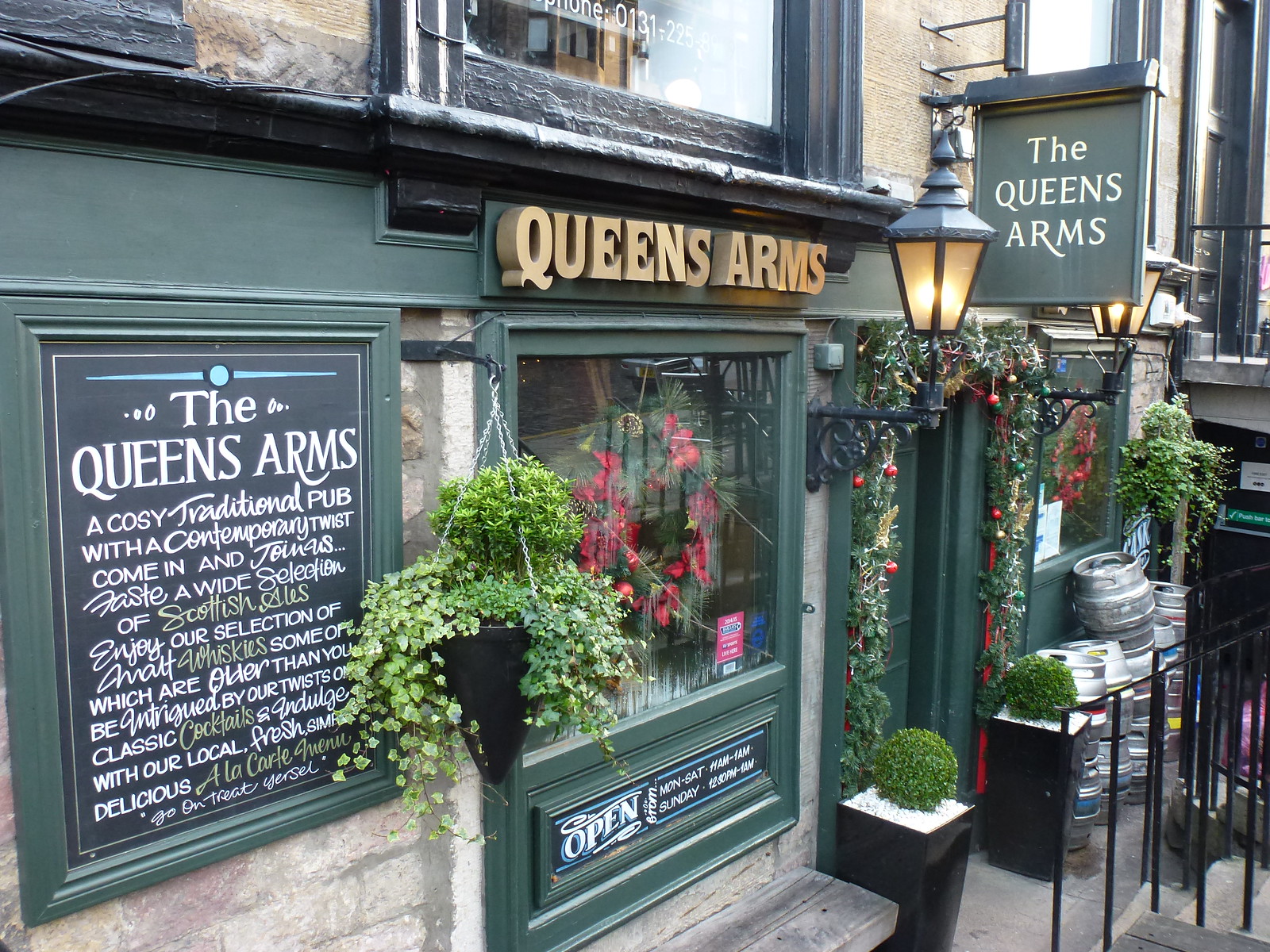The photograph captures the inviting exterior of the Queen's Arms, a cozy traditional pub with a contemporary twist, likely situated in England or Ireland. The pub's name, "Queen's Arms," is prominently displayed in a gold font on a green awning and repeated on various signs. The facade features a charming blend of green wood and whitish brick, with a dark green sign framed by a lighter green border detailing the pub's offerings. Flower pots and a window adorned with a wreath add to the quaint ambiance, while an old-fashioned light fixture illuminates the entrance. Patrons are welcomed with a chalkboard that reads, "The Queen's Arms, a cozy traditional pub with a contemporary twist. Come in and join us. Taste a wide selection of Scottish ales. Enjoy our selection of whiskeys, some older than you, and savor our twists with local fresh produce." The small entrance is accessed via a short flight of stairs with wrought iron railings, and nearby, a stack of beer kegs adds to the charming authenticity of this inviting pub.